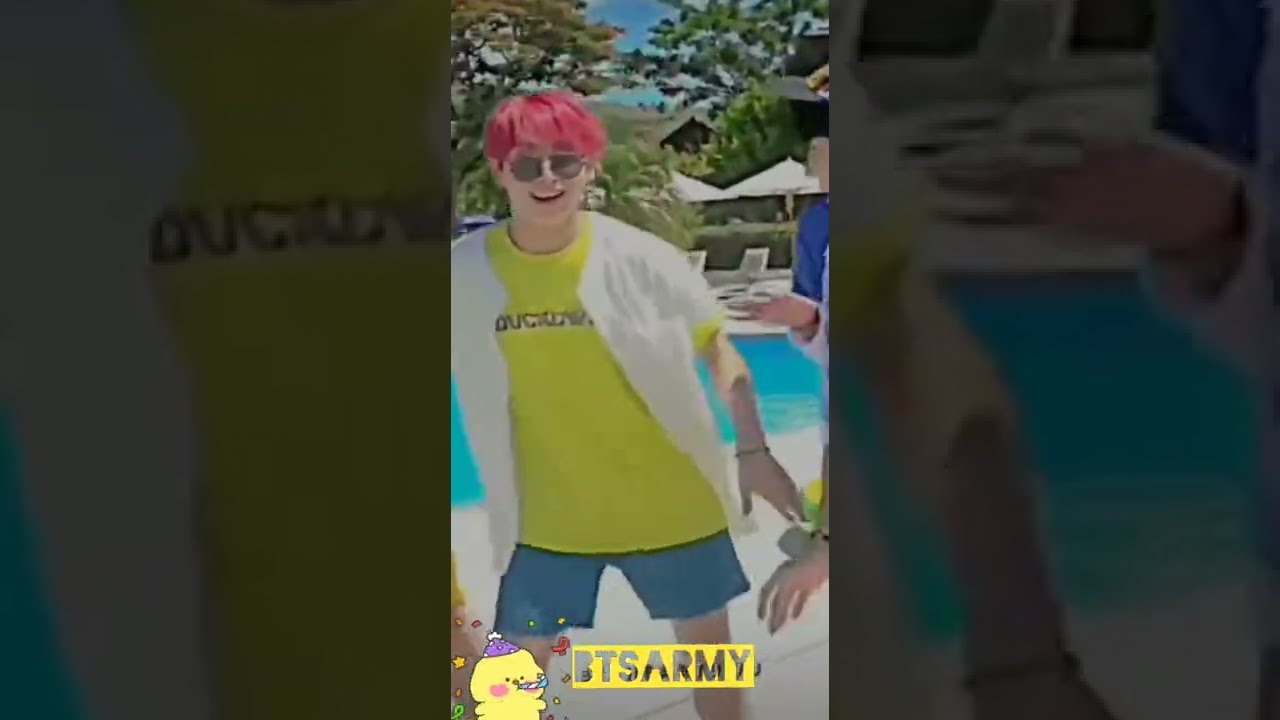The image captures a social media video screenshot divided into three parts: a central image flanked by zoomed-in sections on the left and right. The entire visual forms a rectangle with longer top and bottom dimensions compared to the sides. Dominating the center, an individual is featured with distinct details: pink hair, metallic-framed black sunglasses, and an open white short-sleeve button-up shirt revealing a neon yellow t-shirt with black writing, partially reading "Duckworth." The ensemble is rounded off by blue swim trunks. 

His beaming smile exposes the top row of his teeth. Stenciled at the bottom of the central image is a yellow rectangle bearing the text "BTS ARMY" in black font. In the bottom-left corner, a small yellow chick cartoon with a party hat and confetti around it adds a playful touch. The vivid backdrop includes a bright blue swimming pool, beach umbrellas, lawn chairs, a blue sky, and distant trees.

The left zoomed-in section primarily shows parts of his white shirt and yellow t-shirt, while the right section focuses on his arm adorned with a bracelet, a hand from another person, the pool, and surrounding chairs.